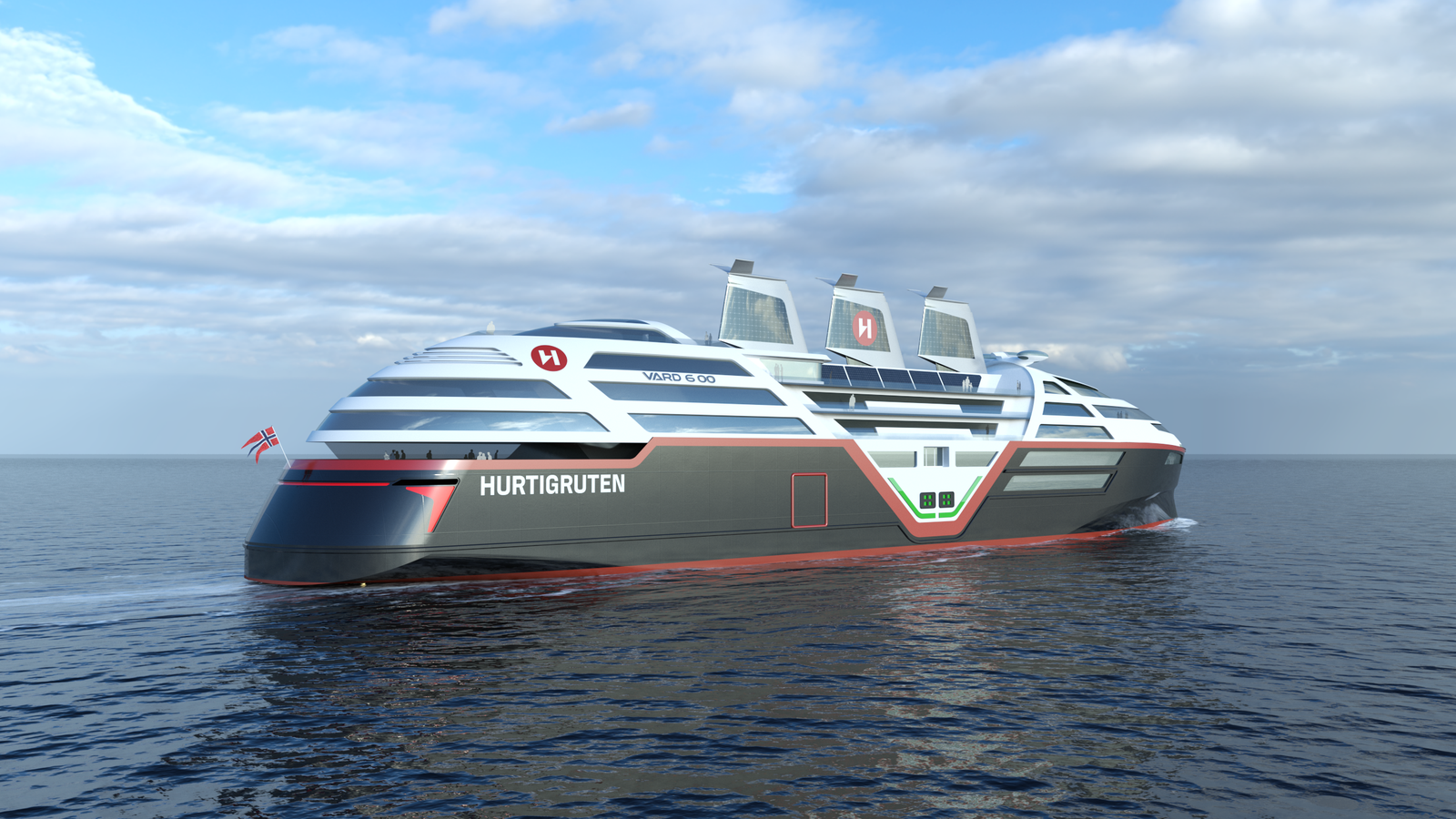This image depicts a large cruise ship, named "Hurtigruten," far out at sea under a cloudy sky. The ship's hull is painted dark gray and outlined in red, with the upper decks featuring a white color adorned with numerous blue-tinted windows. The vessel is centrally positioned in the image, traveling from left to right. A distinguishing feature on the ship is a large logo, a red circle with a yellow "H." Additionally, the ship flies a red and blue flag, resembling a Scandinavian flag, possibly symbolizing its Norwegian origin. The calm, dark blue ocean contrasts the ship's vibrant colors, and a small text reading "Varg and Company" can also be seen. There are three smokestacks on the top center of the ship, and figures, possibly passengers or crew, can be observed standing on one of the lower decks.